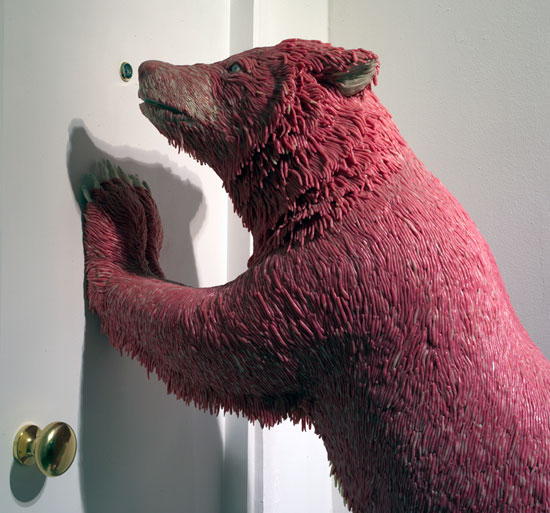This image features a computer-generated, red bear, reminiscent of Paddington, prominently positioned at the center. The bear, with its wet, stringy fur that is almost Play-Doh-like in texture, displays distinctive white patches around its ears, mouth, and front paws. Pressed against a white door with a circular peephole, the bear leans forward, cupping its paws around the opening as if peering through it. To the bottom left of the scene, a gold doorknob can be easily spotted. The backdrop includes a white wall situated at the top right of the image. The bear's eyes are a notable black, and its shadow is cast onto the door, adding depth and realism to the scene.